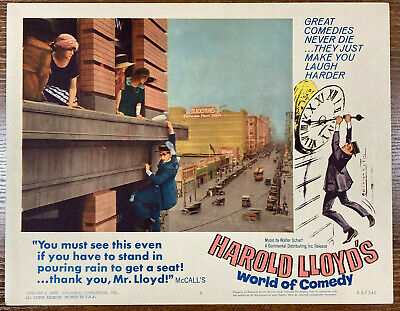The image appears to be a vintage advertisement for Harold Lloyd's "World of Comedy." The poster is in landscape orientation with a cream background. In the lower right-hand corner, it prominently says "Harold Lloyd's World of Comedy" in pink and blue text. Above that, there are inscriptions mentioning music and additional handwriting that is difficult to decipher.

In the top right corner, the text reads, "Great comedies never die... they just make you laugh harder." Below this text is a drawing of a man in a dark suit and hat, hanging from the minute hand of a Roman numeral clock. The clock face has a yellow spot behind it.

The main visual element of the poster, which takes up a significant portion of the upper left, depicts a city scene. Two women, both wearing hats, look out of large windows on a building. Beneath them, a man in a blue suit is hanging by one hand from the ledge. The image captures the bustling city life below, with cars visible on the street.

In the lower left-hand corner, dark blue text reads: "You must see this even if you have to stand in pouring rain to get a seat! ...Thank you Mr. Lloyd." Below this quote, the word "McCall's" is visible, indicating perhaps a publication or endorsement.